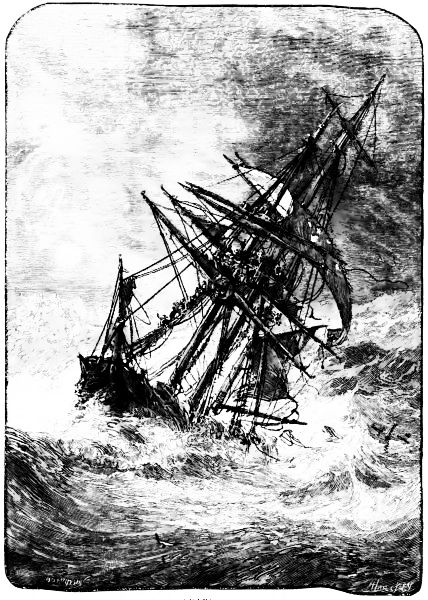This is a black-and-white drawing that looks like it was done with either a pencil or pen, possibly even charcoal, and it appears to be photocopied from a book. The vertical artwork features a large nautical ship caught in a violent storm at sea, positioned centrally in the image. The ship is dramatically leaning towards its port side, almost as if it's on the verge of capsizing due to the fierce waves. These waves are crashing relentlessly against the ship's hull, partially obscuring it. While it’s hard to tell whether the far-right edge of the image shows more waves or rocks, it adds to the chaotic scene. Although some sails have been furled, a few remain, straining under the turbulent conditions. There is an indistinct signature in the bottom right corner, suggesting the work of an artist. This meticulously detailed illustration conveys a sense of impending disaster, almost like minutes before a tragic boating accident.